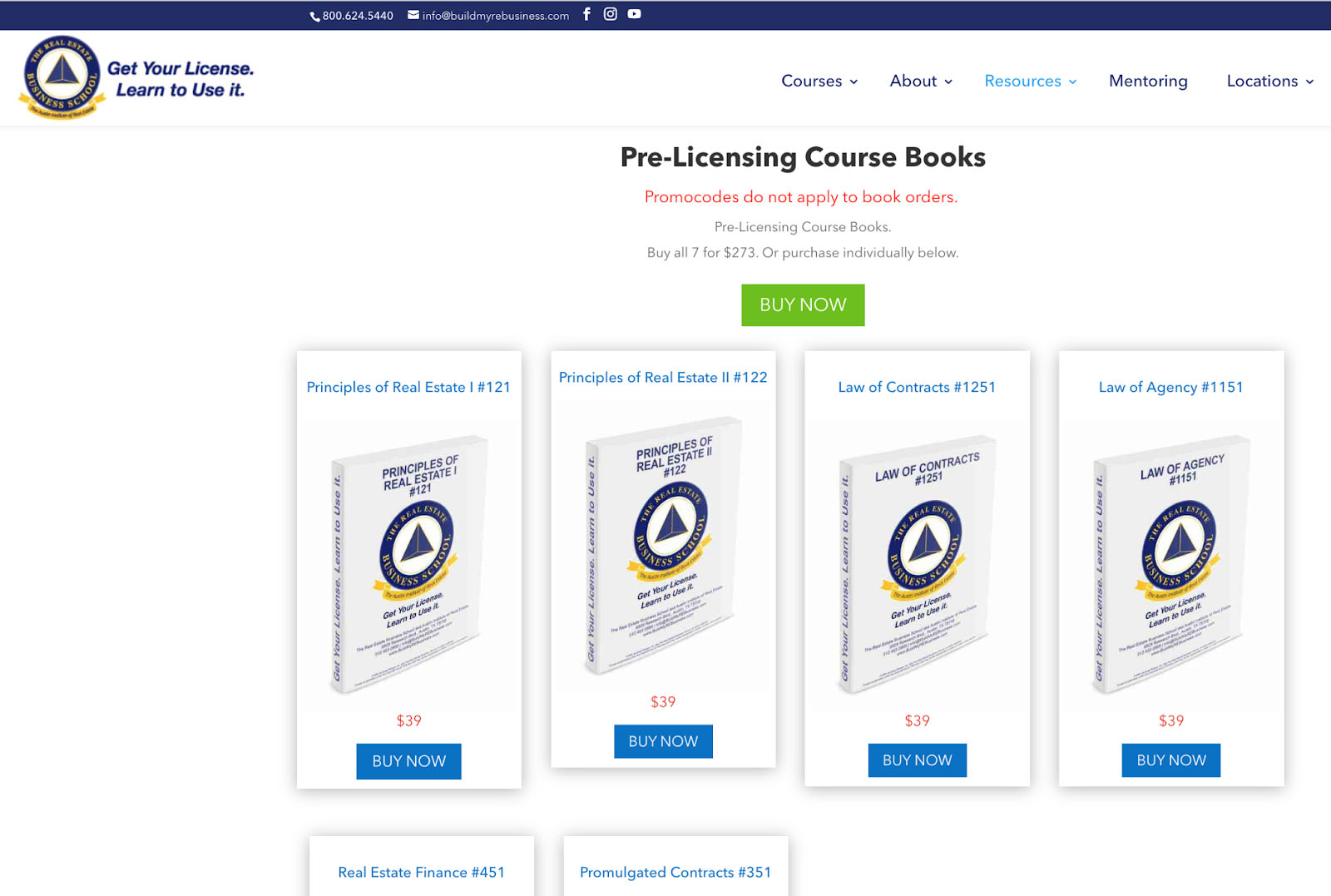The image features promotional material for a pre-licensing course. In the upper left corner, there is a circular logo with a blue edge and a white center, within which is a smaller blue square. The blue edge contains text that is difficult to discern but appears to be associated with a business school. Above this logo, a horizontal blue line includes contact information: a phone number (800-624-5400), an email address (info@buildmybusiness.com), and icons for Facebook, Instagram, and YouTube. To the right of the logo and contact information is a menu that lists options such as Courses, About, Resources, Mentoring, and Locations. Below these elements are four pre-licensing course books meticulously lined up side by side, each displaying a price, ready for prospective students to view and purchase.